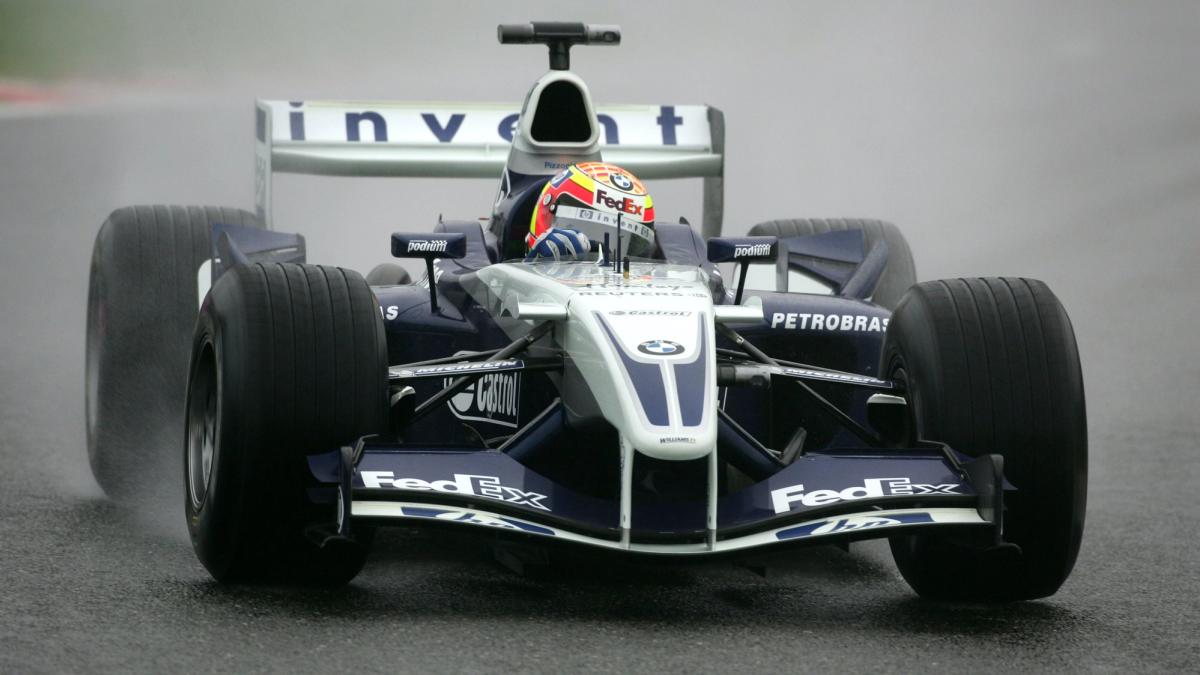This detailed photograph showcases a Formula One racing car, vividly captured mid-race. The car, primarily dark blue with white accents, bears the BMW symbol prominently on its front nose and features the word "FATX" on the front spoiler. The striking contrast continues with the driver's helmet, which is a vibrant mix of red, yellow, and orange, emblazoned with the FATX logo at the top center. As the car speeds along a rain-slicked track, water sprays dynamically, adding to the sense of motion and intensity. The front tires are noticeably narrower compared to the very large rear tires, underscoring the car's high-performance design. The rear of the car sports a horizontal spoiler with the name "Invent" emblazoned on it. Additional advertisements for brands like HP and Castrol are visible on the car's sides. The overall build is sleek and narrow, emphasizing its streamlined nature for optimal speed, with minimal padding around the driver, reflecting the high-stakes world of Formula One racing.